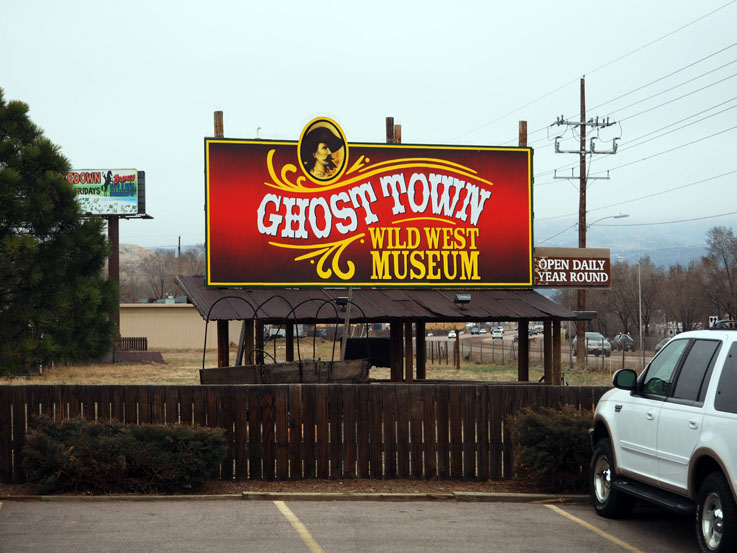This color photograph, though slightly faded, captures a panoramic view of a parking lot dominated by a large red billboard advertising the "Ghost Town Wild West Museum." The billboard, centrally positioned and supported by visible wooden beams, features a gradient of dark to bright red hues, with a distinctive curved yellow banner proclaiming "Ghost Town" in white letters and "Wild West Museum" in yellow beneath it. An oval-shaped portrait of a Western figure, flanked by gold flourishes, is prominently displayed above the text.

In the foreground, there is an empty light gray asphalt parking lot marked with yellow lines. On the right side of the lot, a white four-door SUV with a black luggage rack and silver-rimmed tires is parked nose-in toward the rustic, horizontal wooden plank fence that separates the parking area from the field. Below the billboard, a dilapidated covered wagon, stripped of its canvas but retaining its wooden structure and metal bands, adds to the scene's old-west charm. The background reveals hazy, distant mountains, mostly barren trees suggesting late fall or early spring, a secondary billboard, and elements of a small town, emphasizing the rustic and historic theme of the location. A road is visible along the right edge of the image, running parallel to the museum site. This scene is a blend of representational realism, capturing the essence of a bygone era portrayed through a modern lens.